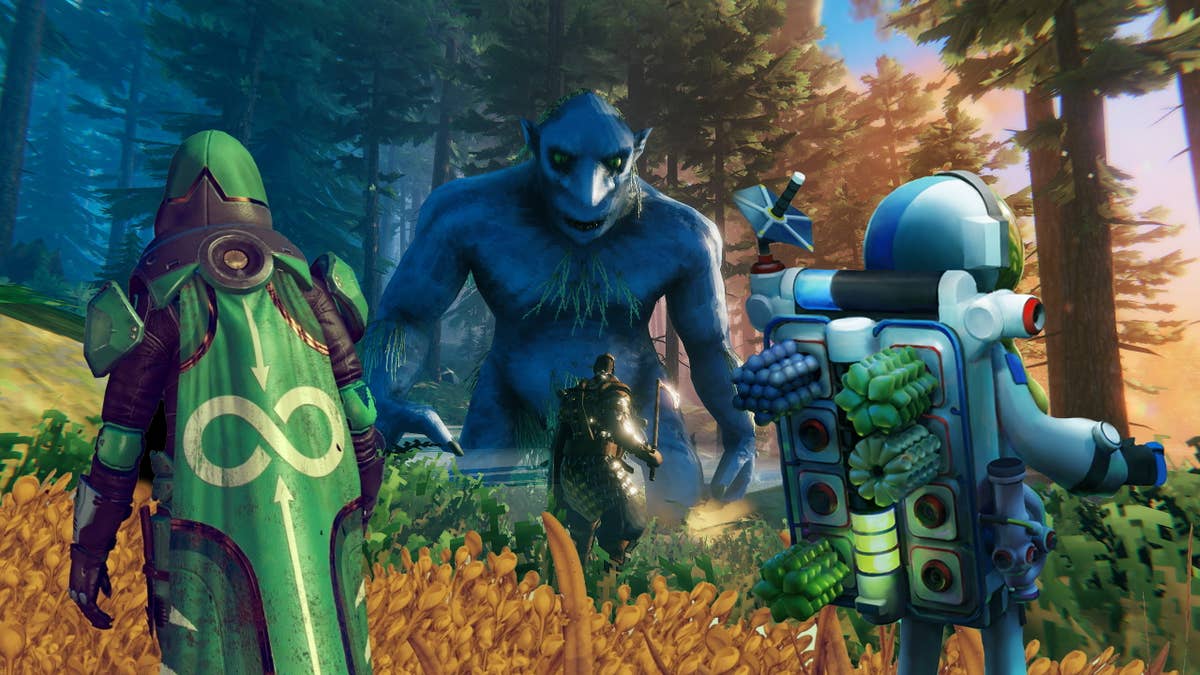The image is a digitally altered screenshot from the video game Valheim, capturing a dramatic scene. In the foreground, there's lush terrain featuring tall green and golden grasses. Dominating the middle distance is a human figure clad in dark steel armor, wielding an axe. This figure confronts an imposing, blue-skinned troll, characterized by its large size, naked and hairy appearance, mean expression, and distinct features including a big nose, green eyes, and pointy ears. The setting is a vibrant forest with towering trees. The right side of the background showcases a sunlit area suffused with green, while the left side is tinted with a bluish hue resembling dusk or shade. Additionally, the image features two digitally inserted characters: a small astronaut from the game Astroneer, positioned on the left, and a guardian from Destiny on the right, each adding an interesting cross-franchise element to the scene. This amalgamation emphasizes the mythical and adventurous atmosphere typical of fantasy video games.